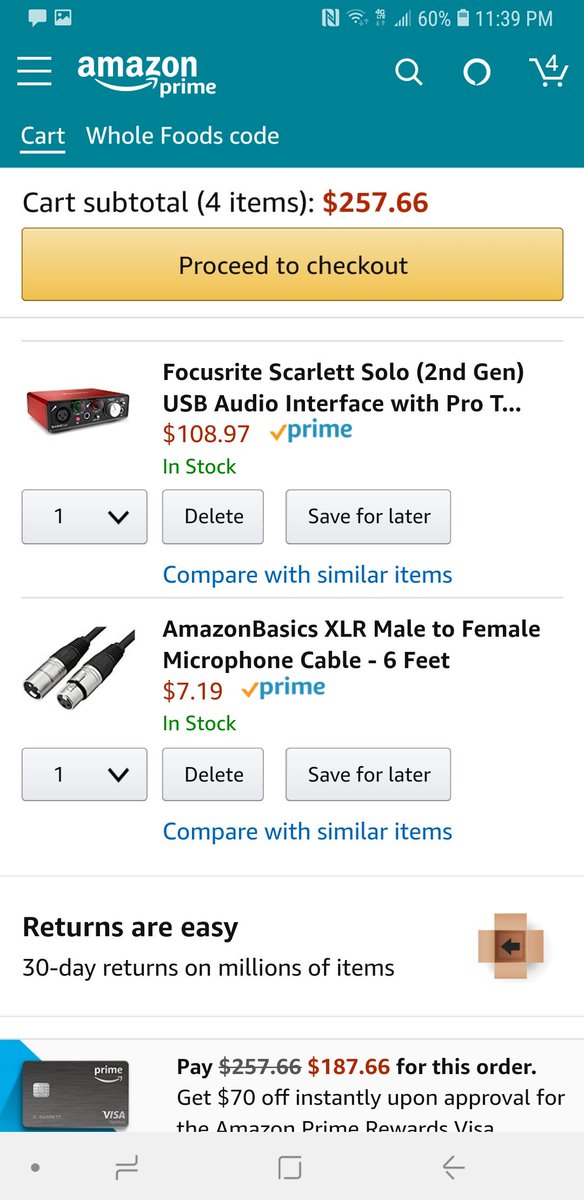In this image, a white background features the Amazon Prime interface. At the top, a blue header includes three white horizontal lines, the Amazon Prime logo, a magnifying glass icon for search, a circle icon, and a shopping cart icon indicating four items in the cart. Below this, the cart section begins with "Your Cart" underlined, showing a subtotal of four items amounting to $257.66. A prominent yellow button labeled "Proceed to checkout" is placed next to these details.

In the main cart area, several items are listed. The first item is the "Focusrite Scarlett Solo 2nd Generation USB Audio Interface with Pro Tools" priced at $108.97, marked as a "Prime" item and noted to be in stock. The quantity is set to one, with options to "Delete," "Save for later," and "Compare with similar items." The second item is an "XLR Male to Female Microphone Cable, six feet," priced at $7.19, also a "Prime" item in stock. Similarly, it shows a quantity of one with the same action options as the first item.

The bottom section of the image highlights Amazon's return policy, stating "Returns are easy, 30 day returns on millions of items," accompanied by an icon featuring a black arrow pointing left. Lastly, a call-to-action message suggests customers can "Pay $187.66 for this order" and get "$70 off instantly upon approval for the Amazon Prime Rewards Visa."

The footer of the image is grey, featuring miscellaneous icons including a dot, two lines, a box, and an arrow pointing left.